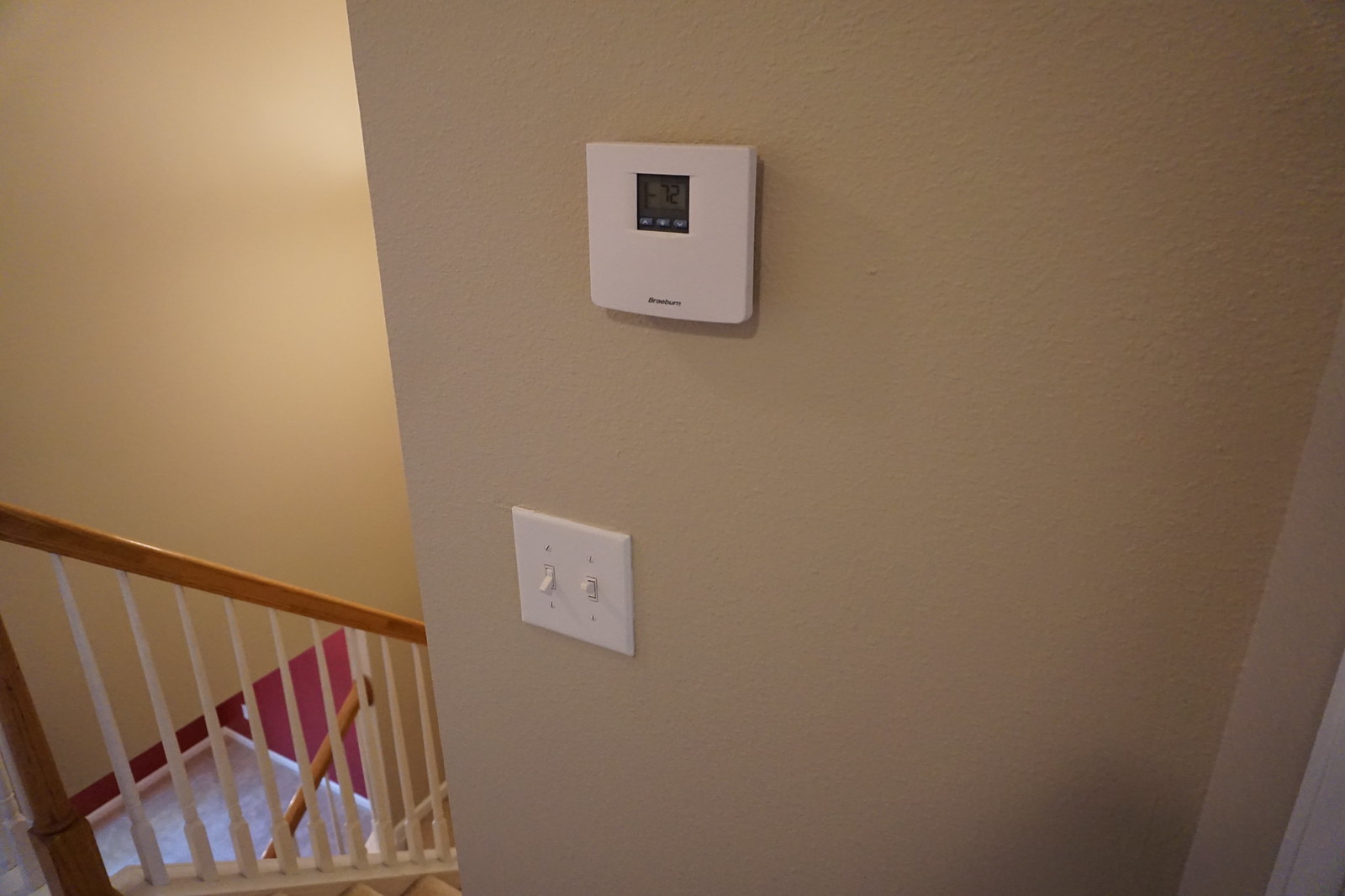The image depicts an indoor hallway featuring a staircase with wooden handrails that are finished with a glossy lacquer. The handrails are accented by white balusters that add a classic touch to the stairway. A brown wall runs alongside the stairs, providing a backdrop that contrasts with the white elements. Fixed to the wall is a white thermostat with a digital readout, neatly displaying the current temperature settings. Adjacent to the thermostat, there is a double light switch plate with two switches; one switch is in the 'on' position while the other is in the 'off' position. The hallway is illuminated by a light source that is located out of frame to the left, casting a warm glow over the scene. Another light switch is visible on the right-hand side of the photo, indicating another access point for controlling the hallway lighting.